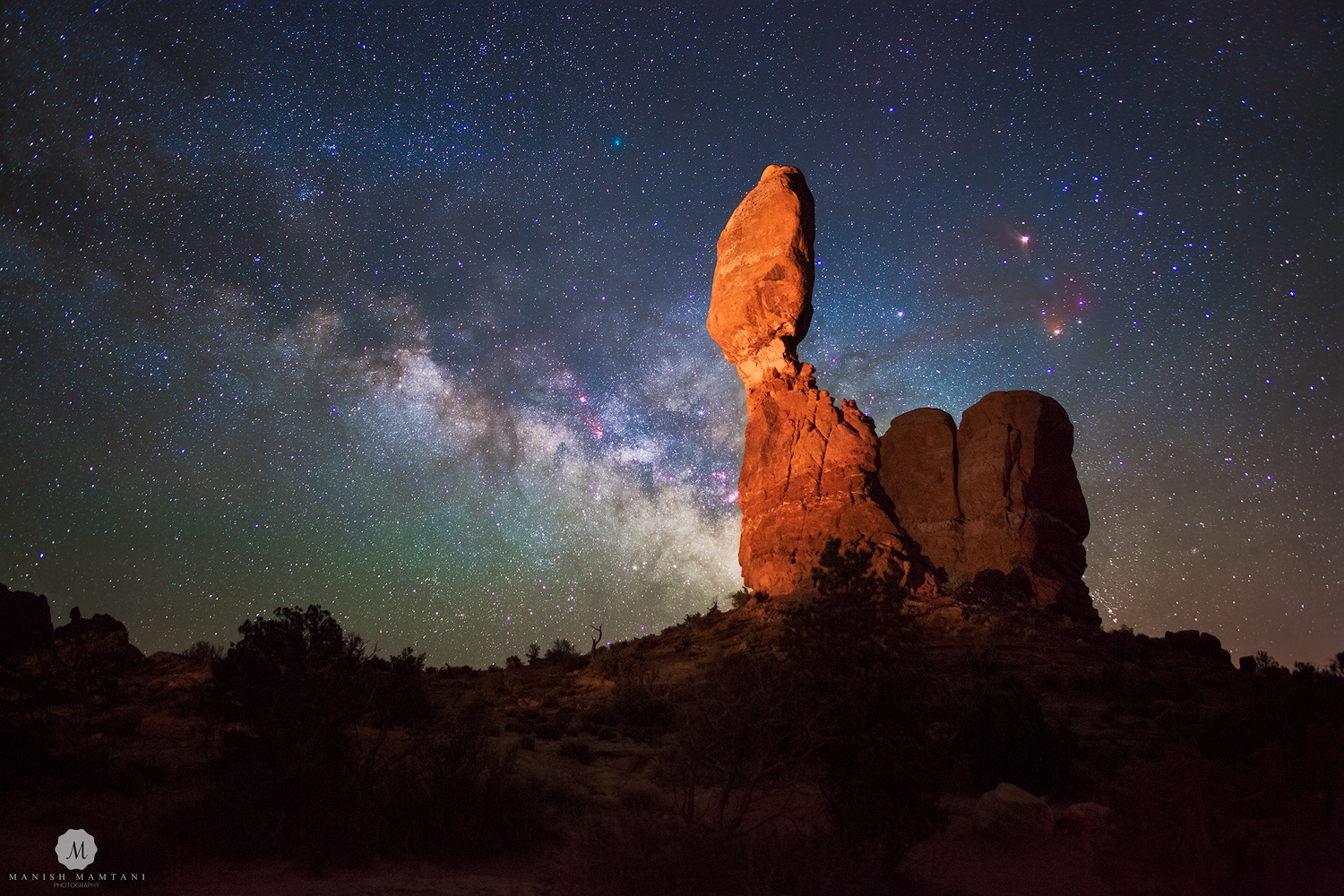In the middle of a serene desert landscape, this nighttime photograph captures a stunning scene under a sky brimming with countless stars of varying brightness. The deep blue night sky transitions into shades of purple and green, giving a hint of the Aurora Borealis in the distance. Dominating the image is a striking rock formation with a prominent, tall red rock standing steadfast in the center ground, defying gravity with its impressive structure. To the right of the rock formation, a shorter, squarer rock can be seen, while the left side of the formation is subtly illuminated by an unknown light source. The foreground reveals the dark land area, dotted with the shadows of sparse desert vegetation and bushes, adding to the rugged scenery. This captivating blend of natural elements and celestial wonders creates an image of profound beauty and tranquility.